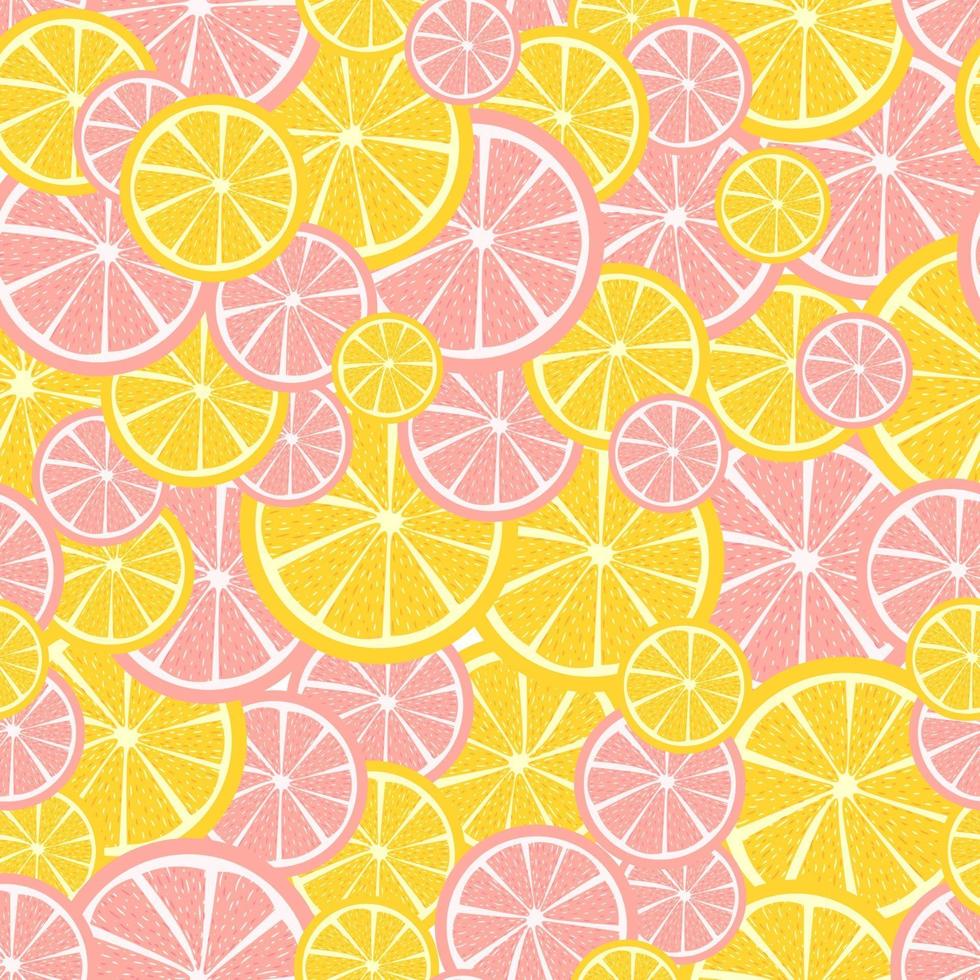This vibrant digital art piece features a wallpaper-style background filled with colorful citrus fruit slices. Predominantly showcasing a mix of oranges and grapefruits, the image is characterized by an array of pink, yellow, and orange slices of various sizes and shapes. These stylized fruit wheels, complete with white segment outlines, are randomly and sporadically dispersed across the entire page, creating a playful and dynamic composition without any apparent pattern or organization. The alternating colors and randomized placement of the citrus slices, resembling lemons, limes, and grapefruit, make for a visually engaging and energetic scene, perfectly suitable for a background or artistic wallpaper swatch.